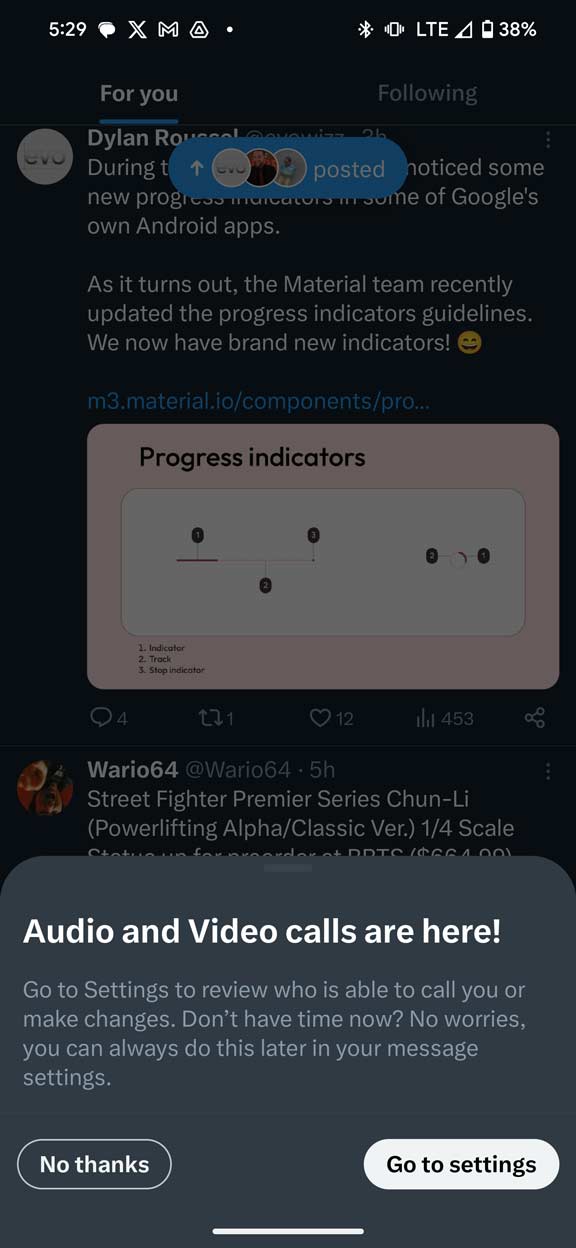In this image, we see a screenshot captured from a cell phone. The upper left corner features a solid black background with white text displaying the time as 5:29. Adjacent to the time, there are icons for messages, Gmail (depicted as a letter "M" with an "X"), and other utilities. In the upper right corner, the battery icon shows 38% and LTE connectivity.

Below this header, there's a blue oblong button with the word "Posted" in white text and three circular icons, one of which appears to say "EVO." In the upper left corner of the main content, a blue underlined link reads "4U," followed by additional, less legible text to the right.

The message body is partially visible, mentioning: “Dylan and I noticed some new progress in some of Google's own Android apps.” It continues explaining that “the Material team recently updated the progress indicators guidelines. We now have brand new indicators” accompanied by a smiley face icon. Below the message, a blue text link reads "m3.material.io/components/pro."

Further down, there’s an expanded section labeled “Progress Indicators” featuring a diagram identifying elements indicated by numbers: 1 - Indicator, 2 - Track, and 3 - Stop Indicator.

Additionally, a tweet by user Wario64 (@Wario64) from 5 hours ago is visible, mentioning: “Street Fighter Premier Series Chun-Li Powerlifting Alpha Classic 1 quarter scale.”